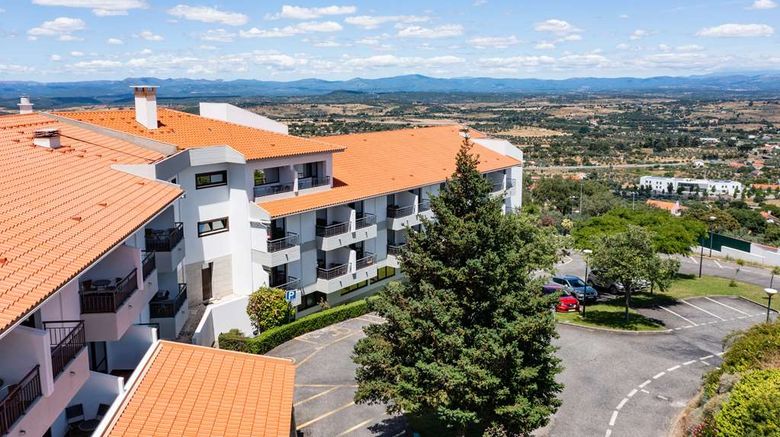This image features an aerial view of a bright white apartment or condominium building, characterized by its terracotta-colored roof and numerous small balconies adorned with black railings. The building is designed with a U-shaped driveway that encircles a large evergreen tree, creating a focal point in the parking lot, which also has several cars parked. In the backdrop, a mountainous landscape is visible, with a mix of other buildings, small houses, and brown plains scattered below. The background vividly showcases a sprawling small town, with one notably long white building, and the scene is enveloped in a blue sky dotted with white, puffy clouds, enhancing the picturesque setting.